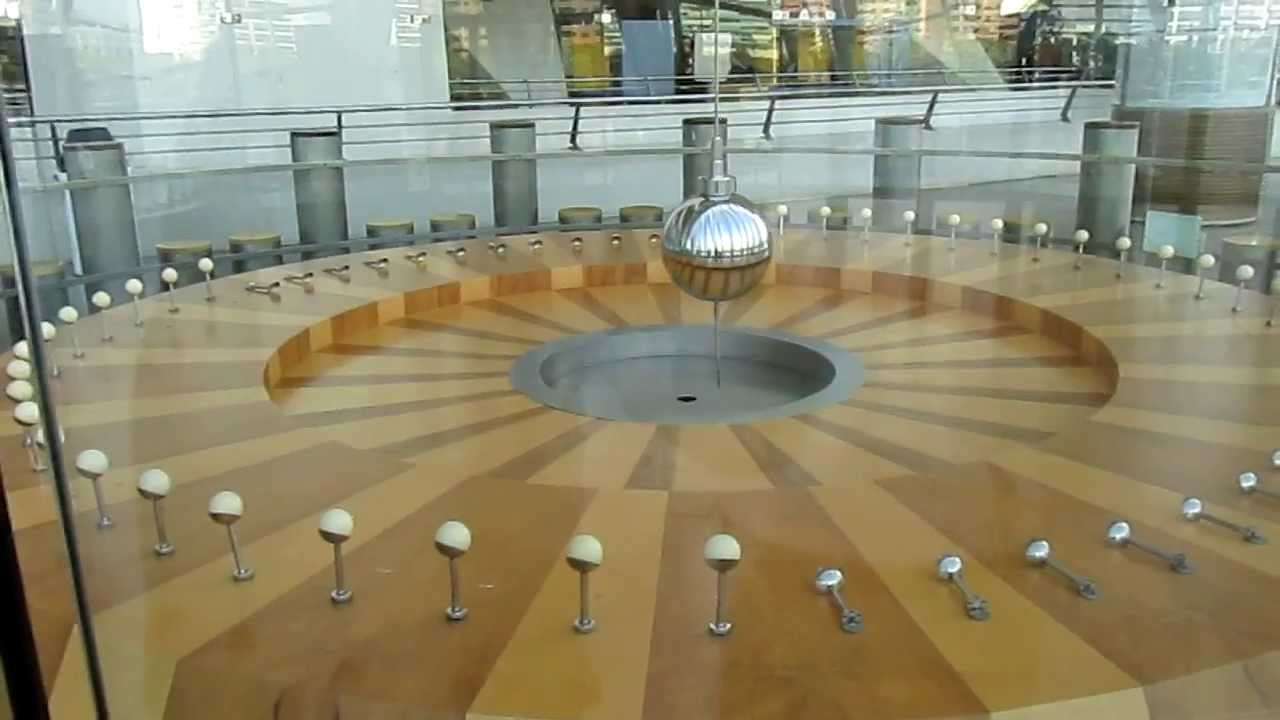The image depicts a detailed museum exhibit featuring a large, circular wooden table arranged in an intricate pattern with light and medium brown slats radiating from the center. At the core of the setup sits a prominent silver ball, likely symbolizing the Earth. Encircling this central sphere are smaller globe-like structures with white tops and brown bottoms, likely representing the moon's orbit around Earth. These globes are attached to steel rods and are positioned both upright and lying flat around the circumference of the table. The exhibit is housed within a space characterized by industrial-type architecture, including white walls, gray concrete slabs, and silver railings. Behind the display, a glass wall accentuates the enclosed, museum-like atmosphere.